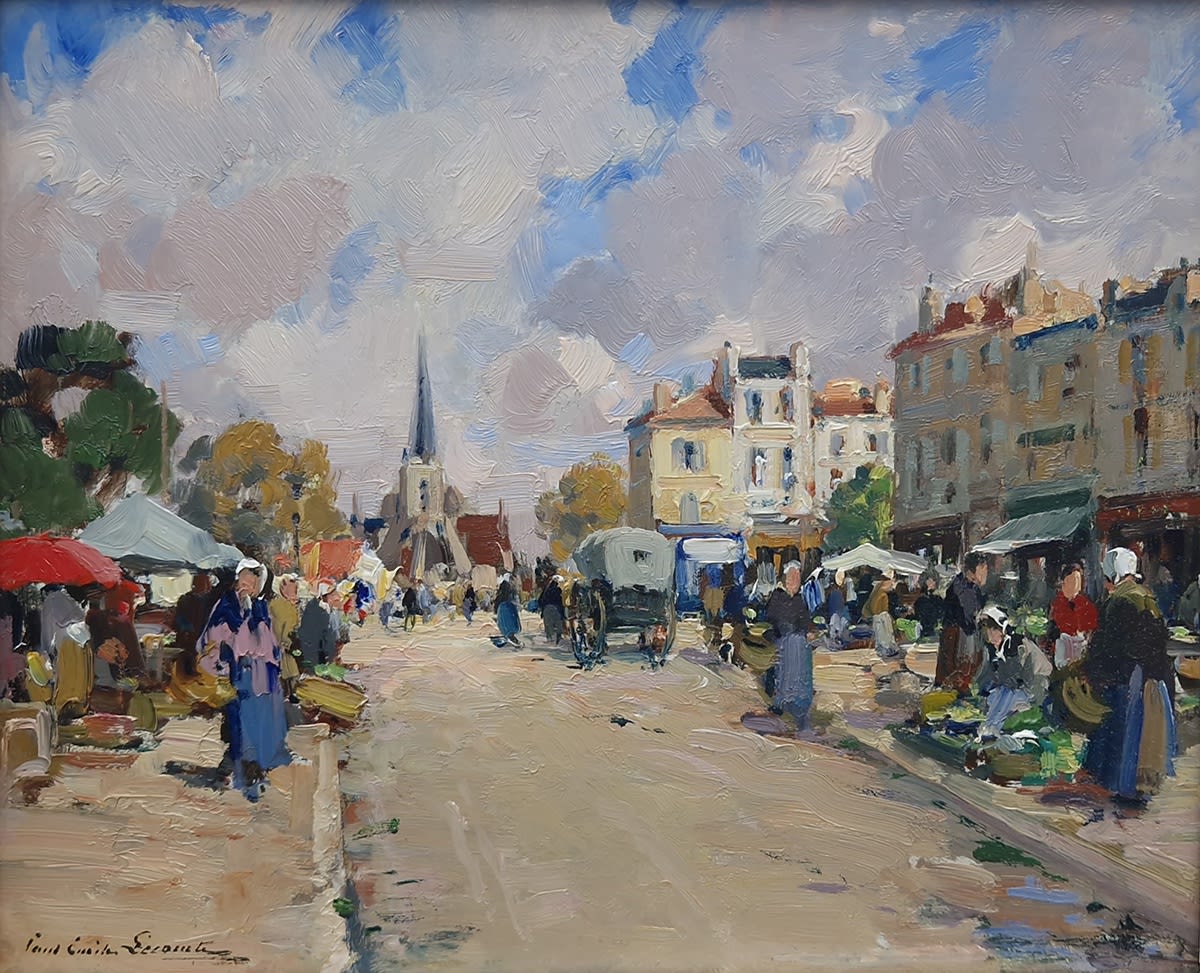In this animated art piece set in a quaint old town, the scene captures a lively street bustling with activity. The road, which appears to be either dirt or slightly decaying cement, runs through the center of the town, flanked by sidewalks on either side. People are gathered along the sidewalks, engaging in shopping and socializing. Many of the women are adorned in white hats, hinting at fashion possibly from the 1700s. The charming peach-colored buildings add a warm, inviting aura to the town. Above, the sky is a serene blue, dotted with white clouds, adding to the picturesque scenery. In the foreground stands a notable church, distinguished by its blue-tipped roof. All elements in the artwork are upright and intact, contributing to the overall harmony and vibrancy of the depicted scene.